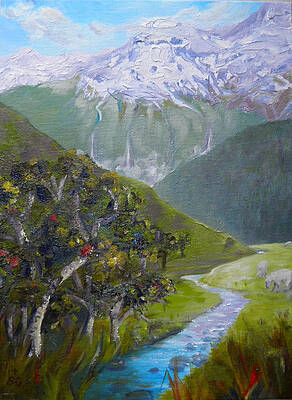The painting depicts a picturesque landscape featuring a meandering brook that flows from the foreground to the background, weaving itself through the center of the image before disappearing around the middle ground. The water transitions from a murky blue to a deeper hue as it curves elegantly from right to left and back again. On the right side of the brook, the foreground showcases verdant grass and a splash of vegetation, possibly highlighting a red bird perched in the very front. This area also includes a couple of rocks and more green grass. To the left, lush green grass is accompanied by trees with brownish-silver trunks, green foliage, and what appears to be red fruit. The left side of the brook rises into green hills, contrasting with the dark shadowy hills on the right, which lead up to grand mountains in the background. These ascending mountains transition from green at the base to majestic, snow-capped peaks crowned with white. The mountain range takes up the top third of the painting, adding depth and grandeur, while fluffy white clouds float in a blue sky above, completing this serene and vertically elongated artwork.